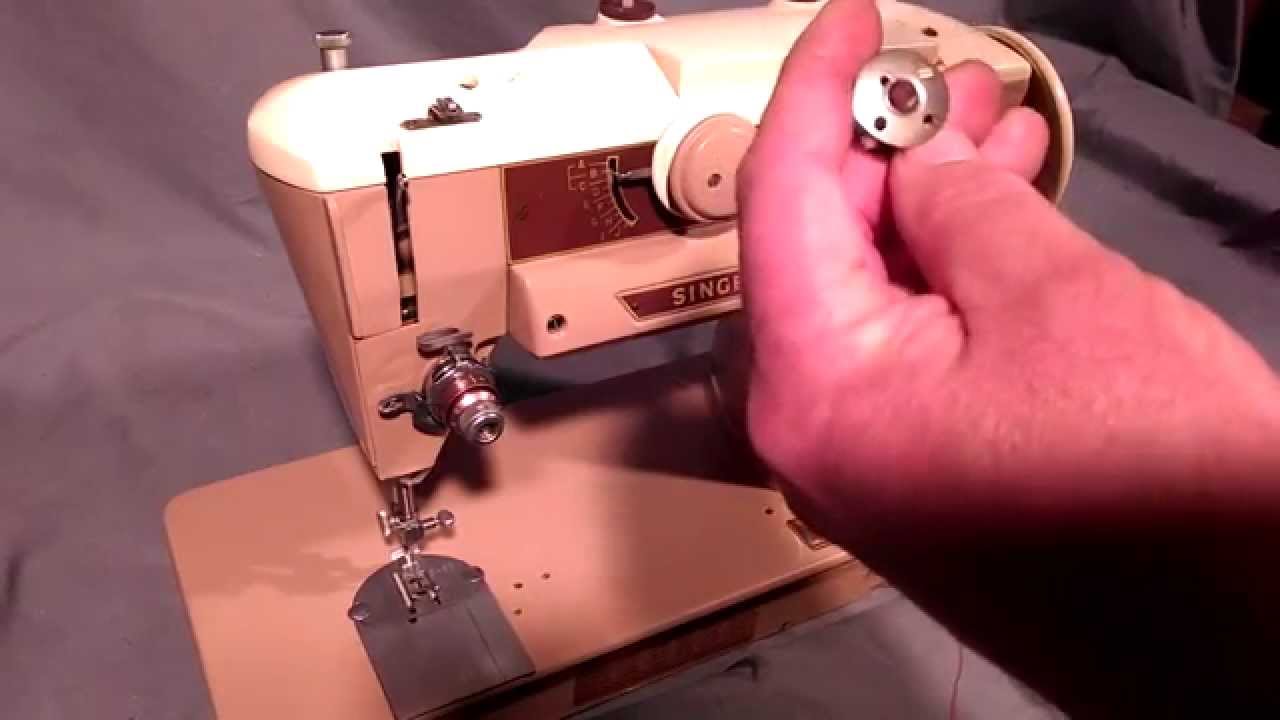The image depicts a vintage Singer sewing machine resting on a gray fabric-covered surface, likely a table or bed. The machine features a classic design with a predominantly beige body accented with reddish-brown and very light brown hues. A white top and the distinctive "Singer" logo are partially visible, although the latter is somewhat obscured by a hand in the foreground. This hand, belonging to a man, is holding a small metal thread bobbin, which has a dull brown shade. The machine's tension control, a reddish round knob, is also noticeable on its frame. The scene is illuminated by an incandescent light source from above, creating bright highlights on the top of the machine and casting subtle shadows underneath it. The overall appearance of the image suggests an old or vintage photograph, emphasizing the classic nature of the sewing machine.